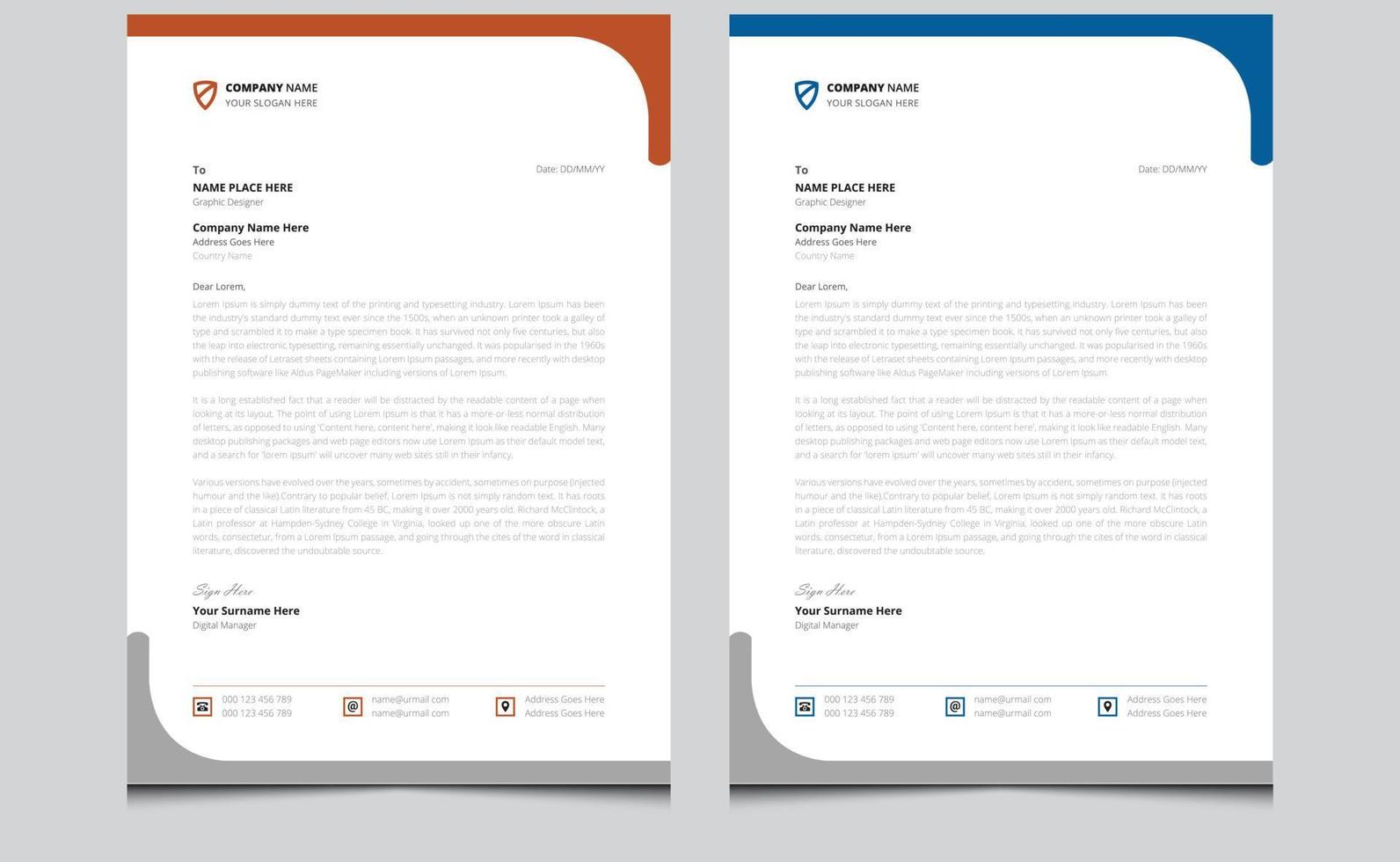This image features side-by-side letterhead templates for a company. Both templates share identical content but differ in color scheme. The template on the left has a dark orange header that spans the top of the page and extends down the right side, covering nearly a quarter of the page. It also has a gray bottom section that runs horizontally and slightly up the left side. The template on the right mirrors this design but uses dark blue for the header and the company logo instead.

Each template contains a company logo that resembles a shield with a cross, placed in the upper left corner. Below the logo, it reads "company name" followed by a slogan, "your slogan here." There is a designated space for addressing the letter to a recipient, specifically mentioning "name place here, Graphic Designer." Further down, it provides sections for the company's name, address, and country, formatted for day, month, and year. The body of the letter includes placeholder text in Latin, serving as a sample of the final layout. At the bottom, there are placeholders for contact information, including phone numbers (represented as 000-123-456-789), an email address, and a physical address. Both templates are designed to show a finished product, demonstrating professional correspondence formatting.